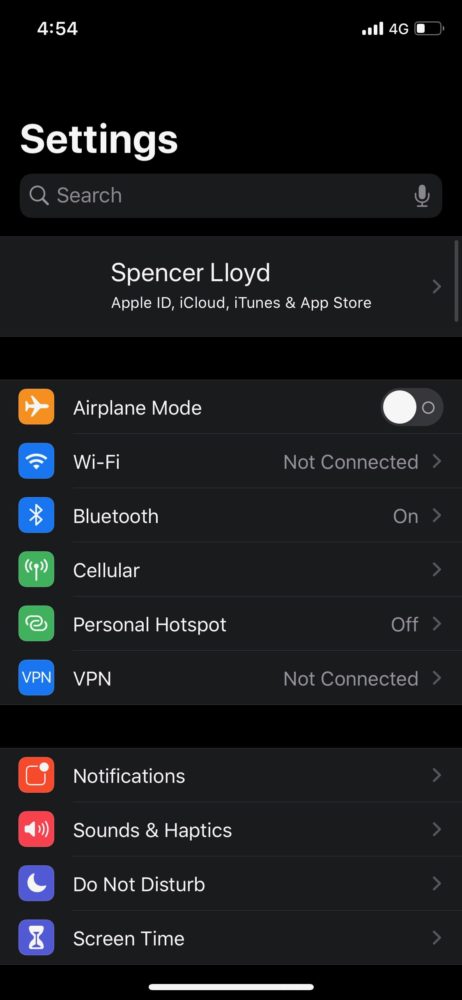**Detailed Caption:**

This is a screenshot of the Settings page from an Apple iPhone, captured at 4:54. The interface has a dark theme, with a completely black to dark gray background and all text rendered in white. The time is displayed in white lettering at the top left corner of the screen. The phone indicates a 4G connection, and the battery level appears to be between 30% to 40%, shown at the upper right corner.

At the top of the page, "Settings" is prominently displayed in large white letters. Below this title, there's a search box for quick access to settings. Further down, a user profile section displays the name "Spencer Lloyd," accompanied by an off-white arrow pointing to the right, indicating a link to more detailed account settings. Under Spencer Lloyd's name, it states "Apple ID, iCloud, iTunes, and App Store."

The settings options are organized in a list format, each item featuring an associated icon to its left:

1. **Airplane Mode:** A toggle option, represented by a white airplane inside an orange square.
2. **Wi-Fi:** Indicated with a blue square containing three lines that symbolize a Wi-Fi signal.
3. **Bluetooth:** Displayed with a blue square featuring the Bluetooth logo.

The list continues with several other options such as Cellular, Personal Hotspot, VPN, Notifications, Sounds & Haptics, Do Not Disturb, and Screen Time. Each of these items has its own respective icon to the left, making navigation intuitive and visually clear.